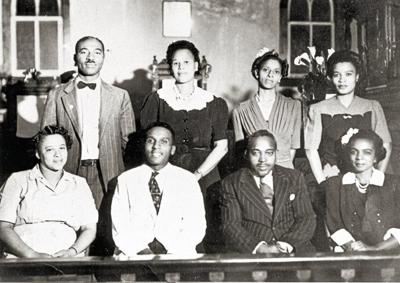This black-and-white photograph, likely from the 1950s, captures a group of eight African-American individuals in a formal setting. The image is in a landscape layout, with the photograph showing some aging and fading. There are two rows of people, four standing in the back and four seated in the front. In the back row, starting from the left, is a man with a mustache, dressed in a pinstriped suit jacket, lighter undershirt, and a bow tie. To his right is a woman wearing a black dress with a white frill around the neck. Next to her stands another woman in a loose-fitting dress that covers her shoulders and reaches down to her elbows. The fourth person in the back is another woman in a dress, though details of her attire are less clear. 

In the front row, seated from left to right, is a woman in a collared shirt with sleeves that reach her elbows. Next to her is a man in a white suit jacket and a dark tie. Following him is a man in a dark pinstriped suit and tie. The last person on the right is a woman in a black jacket with a white collar and sleeves that fall just below her elbows. The background shows windows on each side and a central wall with either a light fixture or a framed item. A railing is visible at the very bottom of the photo, indicating they are inside a large room. Most of the individuals are either looking directly at the camera or slightly smiling.